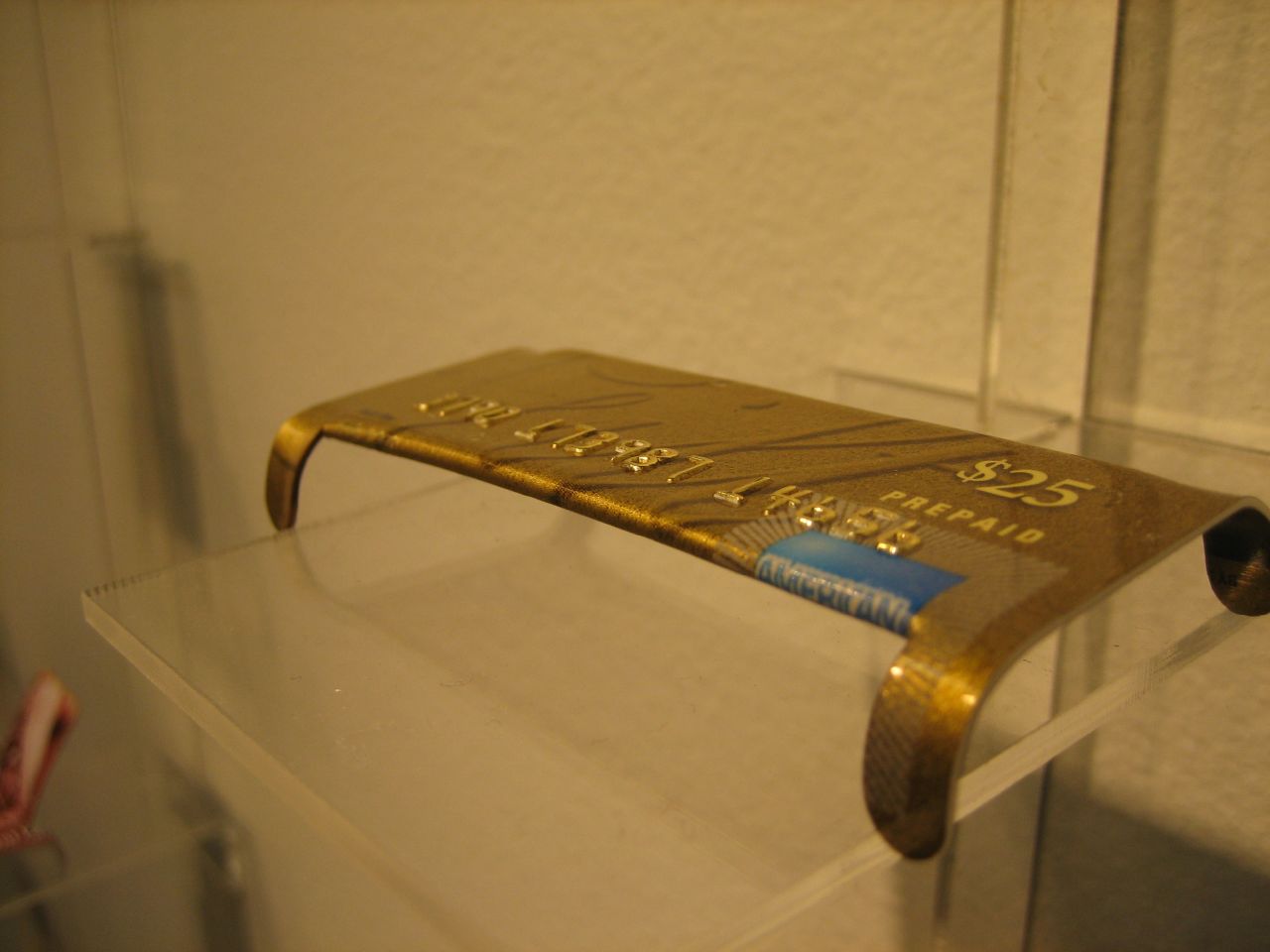The image portrays a creatively transformed American Express $25 prepaid credit card, now fashioned into a bracelet. The golden card features intricate diagonal lines amidst a vibrant gold background and is embossed with the blue American Express logo. The card's edges have been meticulously bent to form a shape that can encircle a wrist, with the very perimeter left intact to serve as the attachment points. This artistic piece is displayed on a clear, wall-mounted acrylic shelf in a retail environment, adding to the aesthetic with its juxtaposition of modern materials and innovative design. The exhibit space has a dark ambiance with a yellowish tone, enhancing the dramatic presentation of this unique sculptural jewelry.